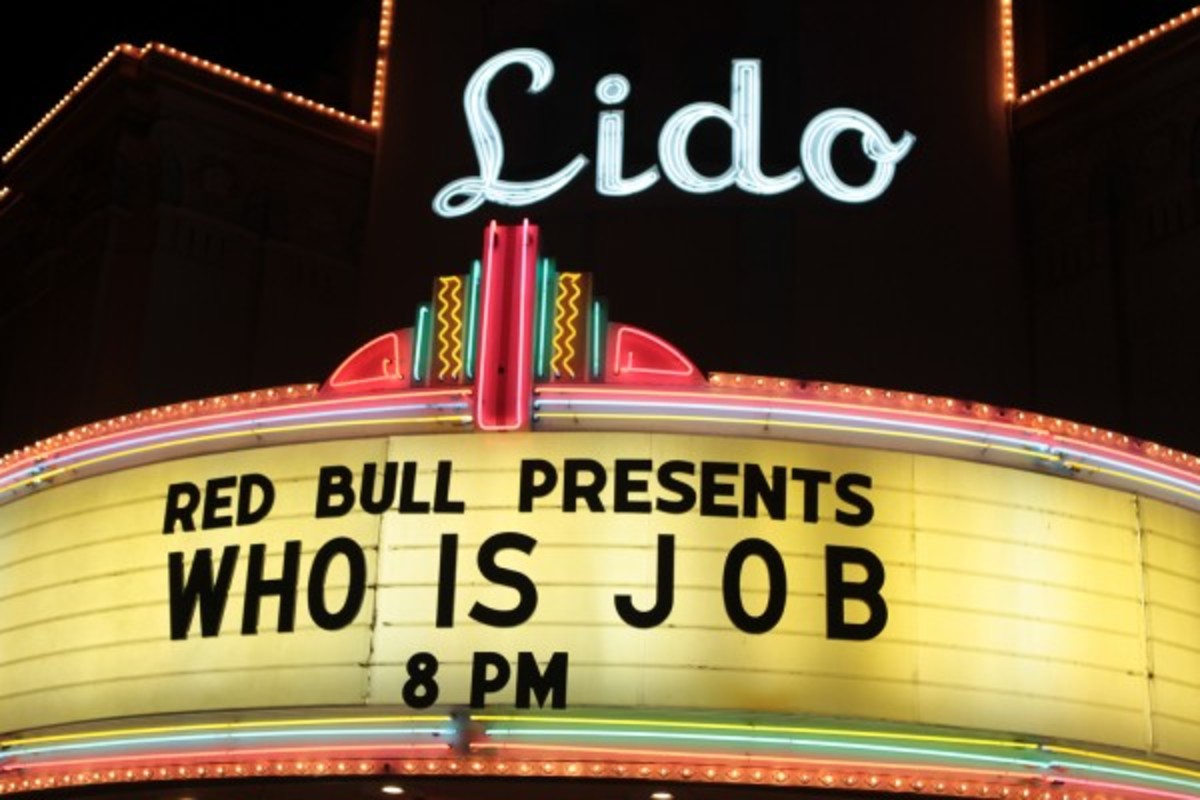This is a nighttime photograph of an old-fashioned theater marquee sign set against a black backdrop. The centerpiece of the sign features the word "Lido" in white neon lights. Flanking "Lido" are jagged lines of orange individual bulbs. Below "Lido," in black capital letters on a white backlit glass panel, it says "Red Bull Presents." Beneath that, also in black, are the words "Who Is Job" and the time "8 p.m." The white strip of text is bordered by thin neon lights in an array of colors—green, lime green, aqua blue, purple, and yellow. In the center of this strip rises a pink neon light. Adjacent to the pink light are two aqua green neon lights, followed by two yellow squiggly lines, and then two more aqua green lights. Red triangles are positioned on either side of this central neon arrangement, completing the intricate and colorful design of the marquee.